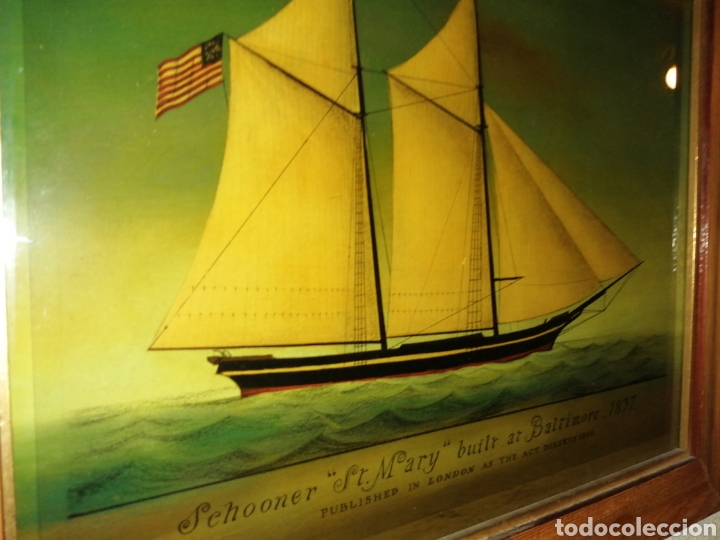The image captures an old artwork depicting the Schooner St. Mary, a white sailing ship with black and red detailing on its hull, built in Baltimore. The vessel, adorned with an early American flag, is shown sailing from left to right across blue waves. The painting is framed in a glossy, brown wooden frame. The text beneath the sailboat is in fancy cursive lettering, stating "Schooner St. Mary, built at Baltimore," though the exact year is somewhat ambiguous, appearing as either 1832, 1837, or 1892 due to legibility issues. Below this, in typewriter-style text, it says "Published in London," but further details are obscured by shadow and the photo’s angled view. A noticeable flash glare to the left side suggests the photo was taken up close, possibly in a museum setting. The bottom of the image features a white stamp stating "To Do Collection."